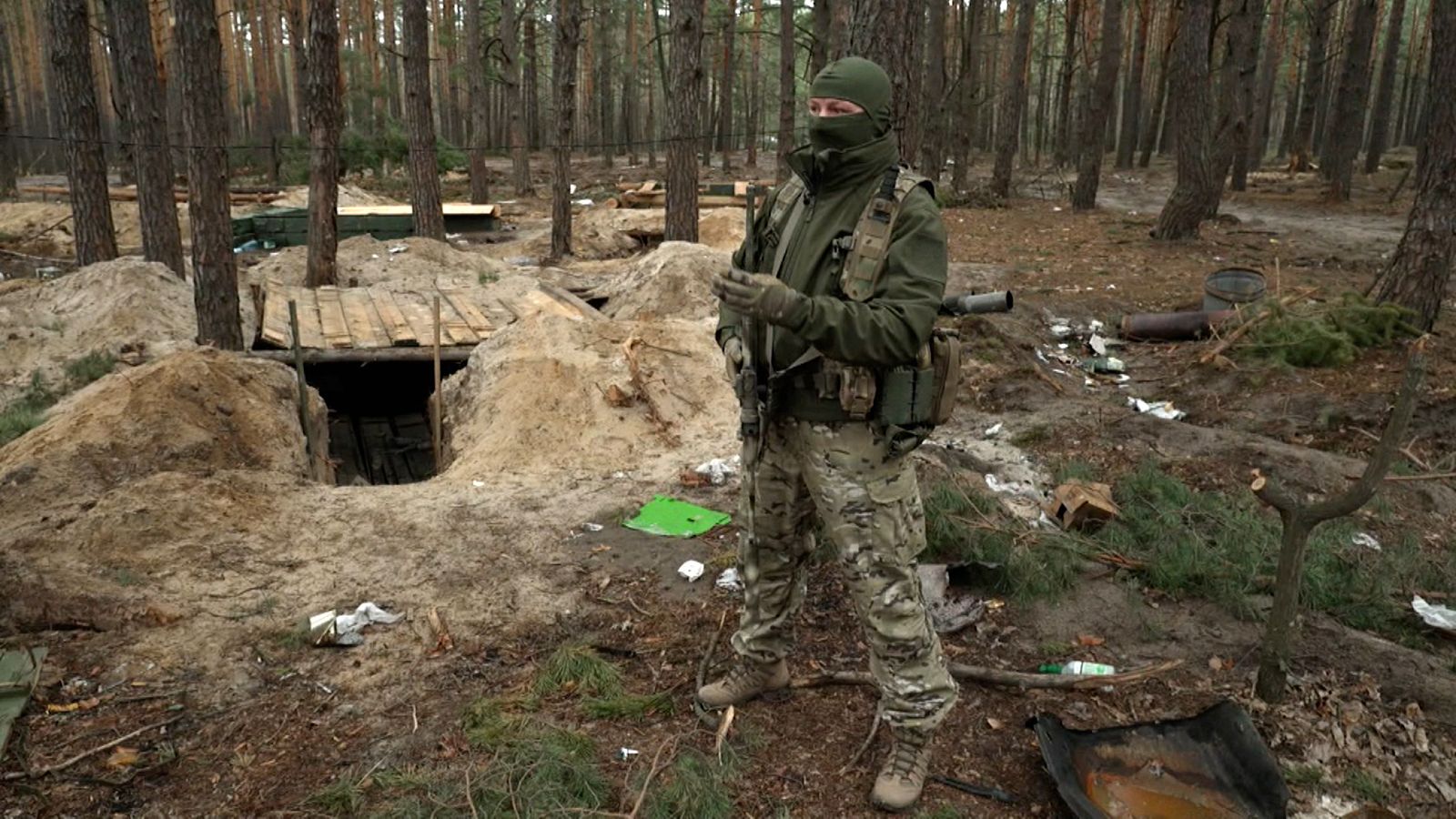In the photo, a figure stands in a dense, wooded area, heavily geared in military attire. The individual, whose gender is indistinguishable, is clad in camouflage pants, brown boots, an olive green jacket, and a dark green face mask that covers their entire face except for the eyes. They are also wearing camo suspenders over the jacket and possibly carrying binoculars or a canteen attached to their left side. The person clutches a rifle, prepared for any situation. Surrounding them, the forest floor is dense with pine needles and littered with various bits of trash and debris. 

To the left, the person has excavated a significant hole in the ground, piling up the displaced earth to form a mound around it. A makeshift wooden roof covers the opening, suggesting the construction of a rudimentary shelter or bunker. Several evergreen branches, still bearing their needles, are scattered, possibly intended for additional coverage and insulation. In the background, similar shelters and sections of cleared trees are visible. The scene conveys a mix of military readiness and survivalist ingenuity amidst the dense, barren trunks and the shaded, underlit forest atmosphere.